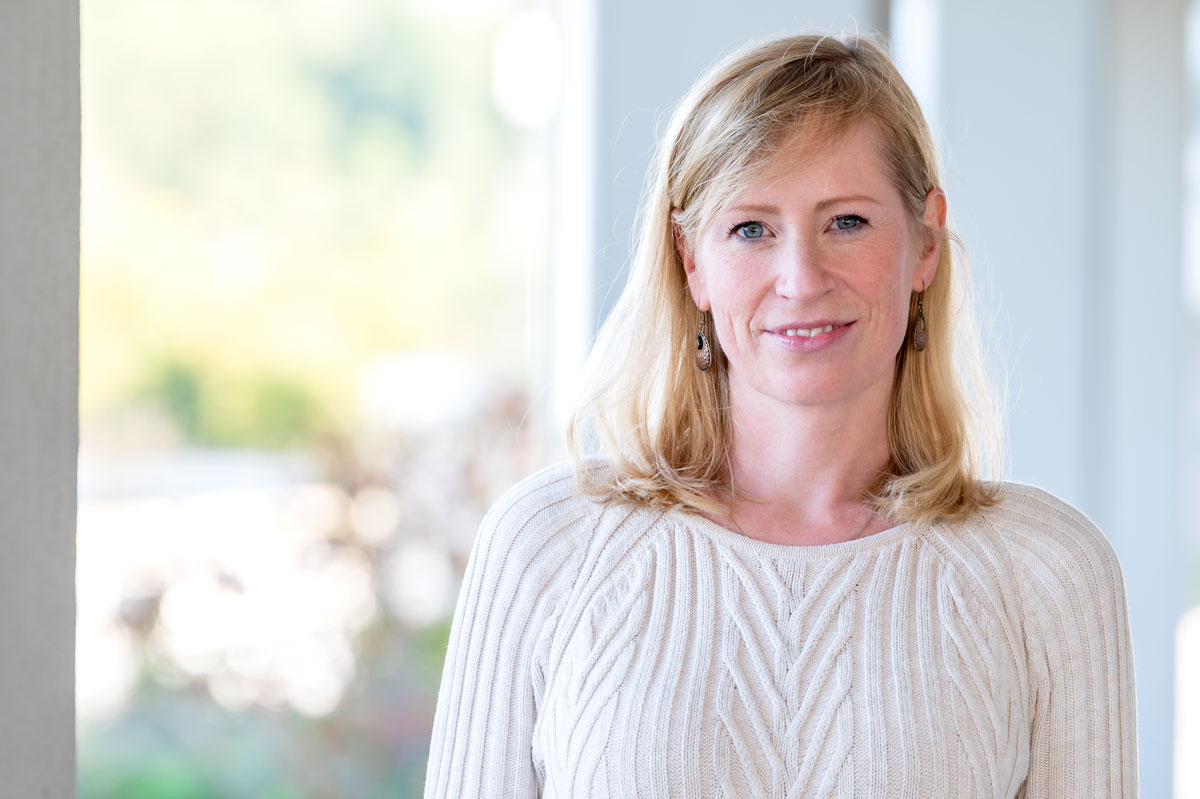This image is a photograph of a woman who appears to be in her 40s, with shoulder-length, strawberry-blonde hair that is parted on the side and tucked behind one ear. Her hair also features swept bangs on one side. She has pale skin, blue eyes, and a slight, dimpled smile that reveals some of her teeth. She is wearing dangly, round, brown earrings and a cream-colored, long-sleeved sweater with a pattern of vertical and crisscrossing lines. Although a necklace is visible, it is mostly hidden under her sweater. The photograph is taken from the chest up, and the background is blurred, featuring indistinct greenery and possibly a window and white wall, keeping the focus entirely on her cheerful expression and demeanor.